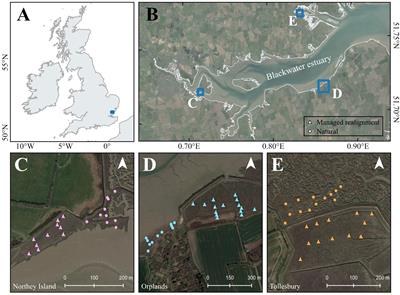The image set consists of five labeled illustrations, arranged with two at the top and three at the bottom, showcasing varied geographical perspectives. Image A, located at the upper left, features a line drawing of Great Britain on a white background with a notable blue dot marking a significant location. To the right, Image B presents a more realistic aerial view of the Blackwater Estuary, depicted in shades of green and blue, identifying waterways and pinpointing the locations of Newt Nesperry Island, Orph Lands, and Tulsbury with corresponding labels in white text. 

The bottom row includes Images C, D, and E, each providing closer, more detailed aerial views of specific areas identified in Image B. Image C, positioned at the bottom left, shows a landscape with vivid green in the upper left transitioning to brown in the bottom right, labeled as Newt Nesperry Island, and features red lights. Image D, in the center, reveals an area marked Orph Lands, with green in the bottom right and brown in the top, and contains blue lights. The final image, E, on the bottom right, offers a detailed view similar to a Google Maps perspective of a predominantly brown land dotted with small yellow triangles, signifying Tulsbury and displaying orange lights. Collectively, these images provide a comprehensive and detailed representation of different geographical and environmental aspects of the same overall region.